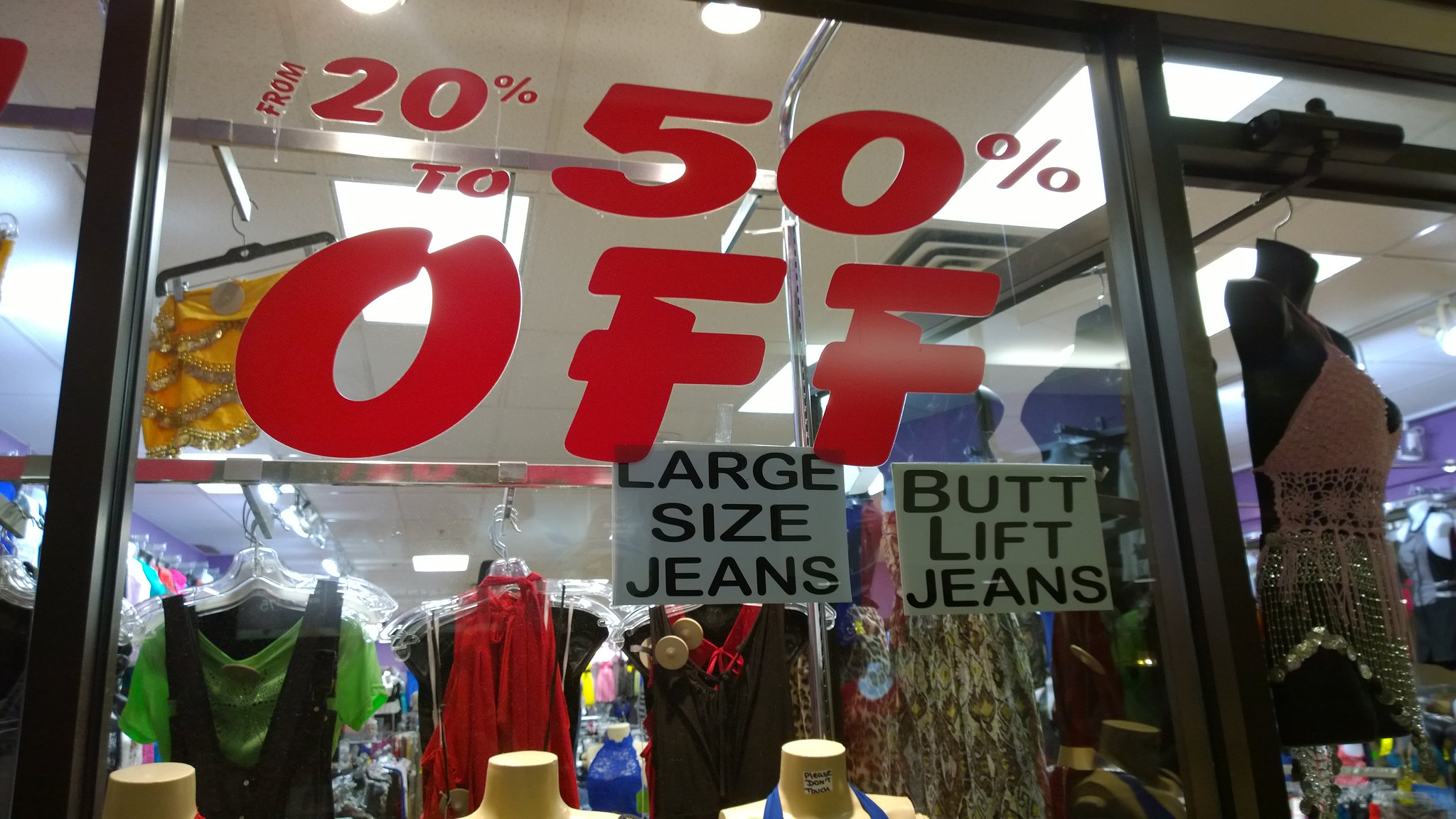This vibrant store window display features bold red lettering announcing, "From 20% to 50% off." Below this, two black and white signs clearly label items of interest: "Large Size Jeans" and "Butt Lift Jeans." The window provides a peek into the store, revealing a variety of garments on clothing racks inside. Prominently hanging behind the letter "O" is a bright yellow skirt adorned with sparkling gold beads. To the lower left of the skirt, a green shirt with black suspenders is noticeable. Moving rightward, a red scarf is draped over a black shirt, which is positioned next to another black shirt with an eye-catching red silk collar. Further to the right, a colorful skirt with an intricate pattern adds a splash of vibrancy to the display. Completing the ensemble, a short, elegantly beaded dress is showcased on a mannequin at the far right.